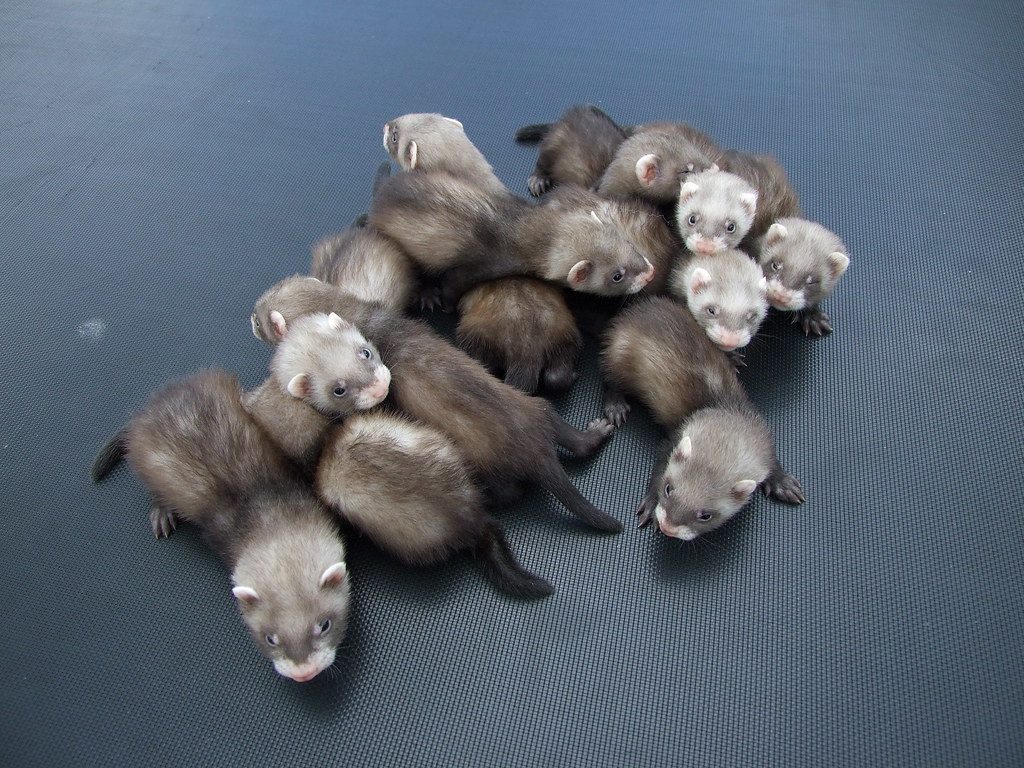This striking landscape-length photograph captures a delightful scene of approximately 10 to 12 young ferrets, closely huddled together and climbing over each other, their playful nature evident. The ferrets, showcasing a mix of gray, brown, and black fur with varying amounts of white on their faces, are sprawled on a textured mat that appears to be black or gray canvas. While most of their faces are pointed in different directions, with some gazing towards the camera and others looking away or hiding, their similarity in patterns and youthful appearances contribute to an endearing and chaotic composition. The background features a dark blue gradient with small ripples, and a subtle light effect in the upper left corner, reminiscent of gentle sun rays, adds an extra touch of warmth to the scene.